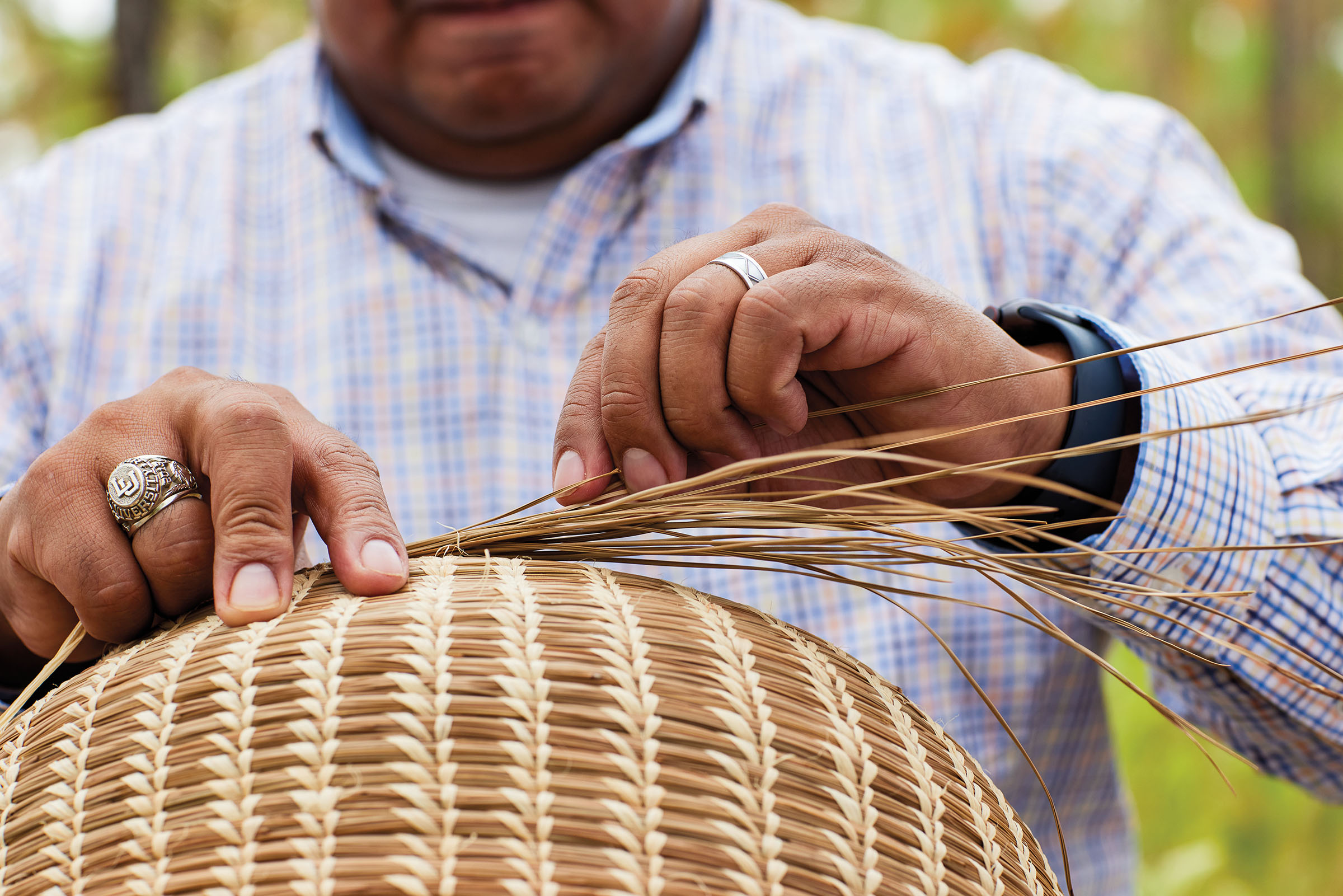A detailed picture shows a husky black man meticulously weaving a wicker basket. The intricate basket, appearing upside down, is being constructed from tan, dried strands resembling dead grass. The man's hands are engaged in an under-over weaving technique. He wears a distinctive ring on his right middle finger, which features a sports emblem with "LU" inscribed on it, in addition to a clasp ring. On his left ring finger, a gold wedding band is visible. His attire includes a long-sleeve shirt adorned with a complex pattern of thin pinstripes or small plaids in shades of light blue, dark blue, purple, orange, yellow, and white, complemented by a white t-shirt underneath. A black-banded watch adorns his wrist. Only his lips, chin, and the thick neck are visible in the frame, emphasizing his focused dedication to the intricate craft of basket weaving.